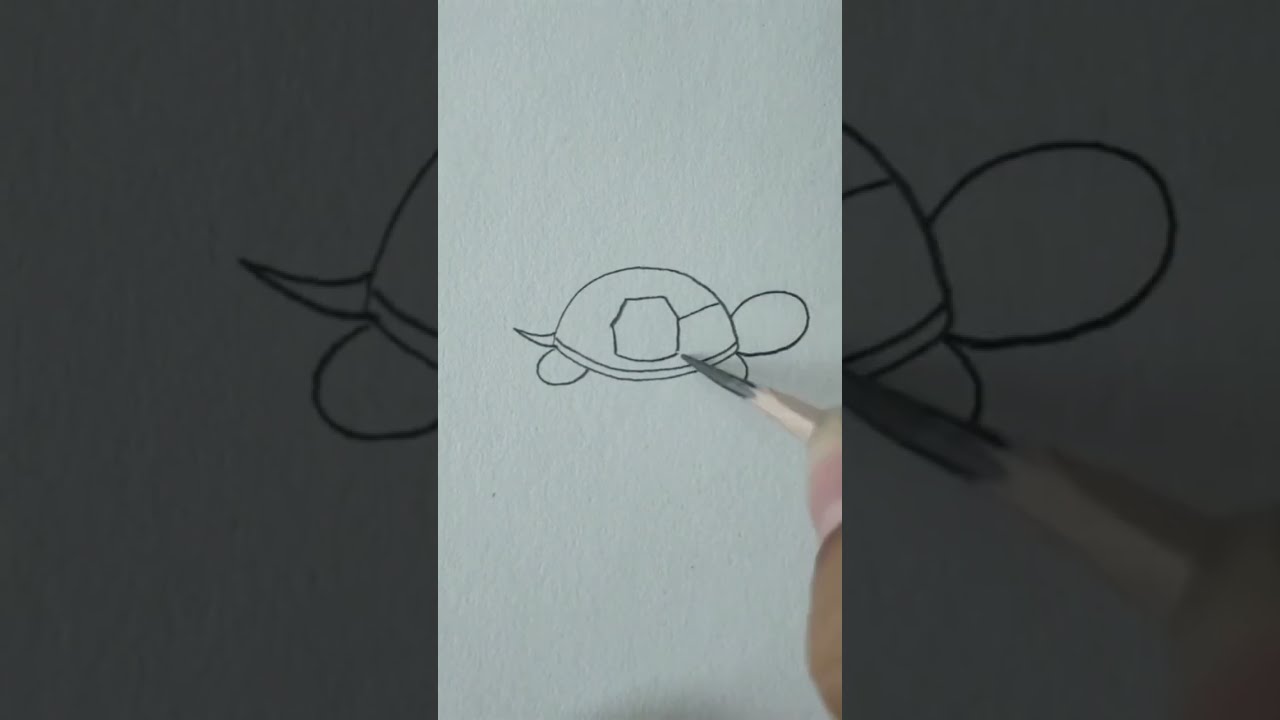In this detailed image, we see a close-up of someone actively drawing a simple, line-drawn turtle on an off-white sheet of paper. The turtle is centered in the image, occupying a small portion of the space with ample white space above and below it. The drawing features the turtle's legs, rough outlines of its head, and an auspicious beginning on the shell, with intricate geometrical shapes being added. Notably, there is no text present on the image canvas. The scene also showcases a pencil with an unusually long, sharp lead point emerging from the bottom right corner, along with a small portion of the artist's fingertip. The background includes a grayed-out, larger rendition of the same turtle image, extending slightly on both the right and left sides, giving the impression of a layered, composite visual. The color palette primarily consists of off-white, gray, tan, pink, and brown hues, suggesting a digital screenshot, likely from a mobile device displaying a TikTok or Instagram live session.